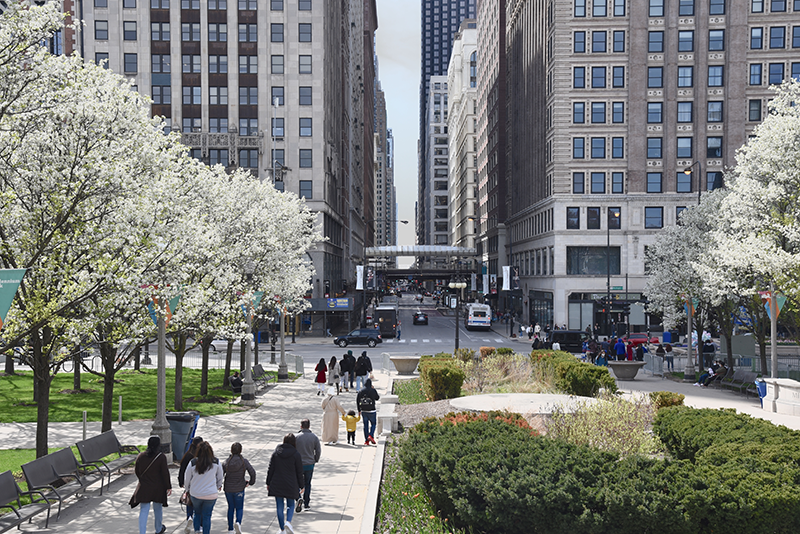The image captures a vibrant spring day in a modern city park. The park is bustling with life, featuring multiple white blossom trees with brown bark lining a busy sidewalk where people are strolling, some holding hands and children in colorful jackets. The park includes scattered gray and black benches mainly placed to the left of the path. Alongside the right of the sidewalk is a small raised circular slab surrounded by green bushes and shrubs. Beyond the park, a city street teeming with cars, buses, and even a UPS truck stretches off into the horizon, flanked by towering gray skyscrapers with numerous light blue windows. The tall buildings on either side of the street are interconnected by a small bridge. The entire scene is detailed with greenery, including numerous trees, green plants, and grass, and is illuminated by the daylight, offering a clear view of the bustling urban cityscape extending to the vanishing point.